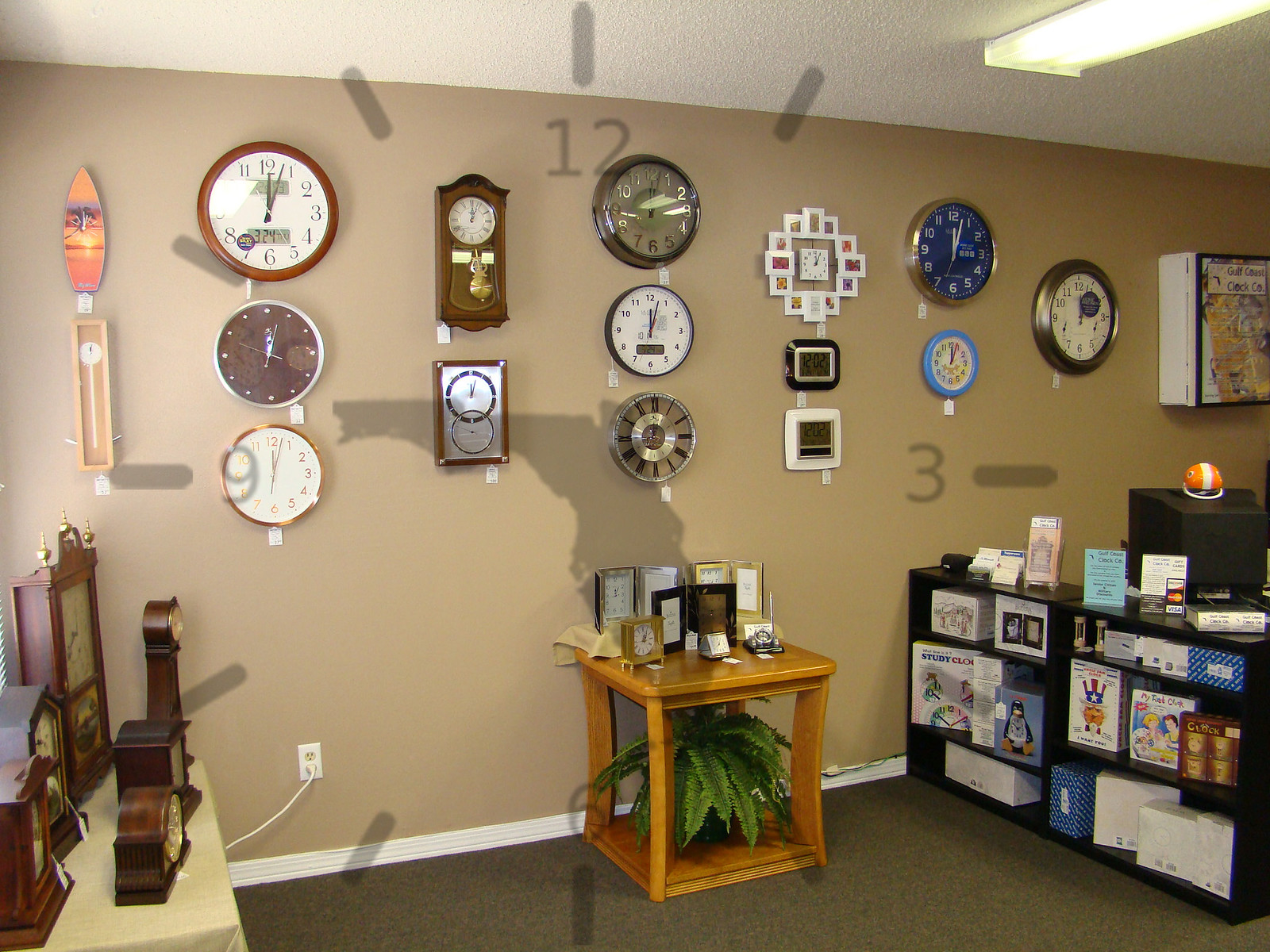The image depicts a room that appears to be a clock store, characterized by an array of diverse clocks adorning the beige walls, each sporting a price tag. The left side of the room showcases a table in the far corner, exhibiting antique wooden clocks. Alongside this table is a visible electrical outlet with a cord plugged into it. Centrally located in the room is a wooden coffee table with square clocks displayed on its surface and a fern plant underneath. On the right, there's an outdated CRT monitor indicative of the mid-2000s, accompanied by a cube-style shelf holding various indistinguishable products. The atmosphere suggests a small, niche shop, perhaps located in a strip mall, emphasizing both practicality and a specific target audience. Various clock designs are evident, ranging from small grandfather clocks to unique, modern ones, including one shaped like a surfboard.